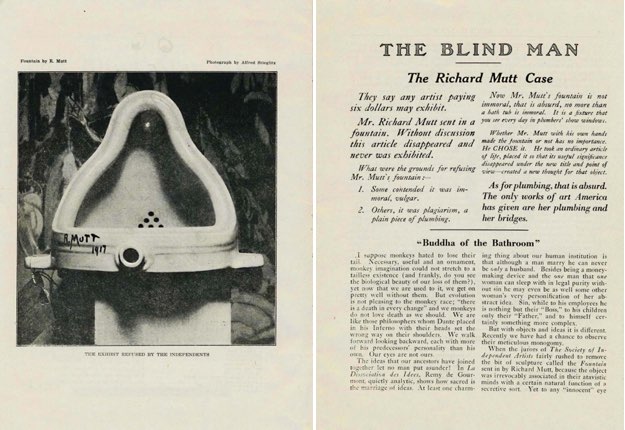This image depicts two adjacent pages from a black-and-white publication. On the left page, there is a photograph of a white urinal, signed "R. Mutt 1917" along its edge, with indistinct background elements. The right page features an article titled "The Blind Man" with a subheading, "The Richard Mutt Case." The text beneath explains that any artist paying $6 may exhibit their work, referencing Mr. Richard Mutt, who submitted a fountain that mysteriously disappeared without being exhibited. The article discusses the varying reasons for its refusal, with some arguing it was immoral or vulgar, and others calling it plagiarism or merely a piece of plumbing. Below this, there is another write-up titled "Buddha of the Bathroom." The text is arranged in two columns, providing a detailed account on the debated fountain and the controversial decision surrounding its exhibition.